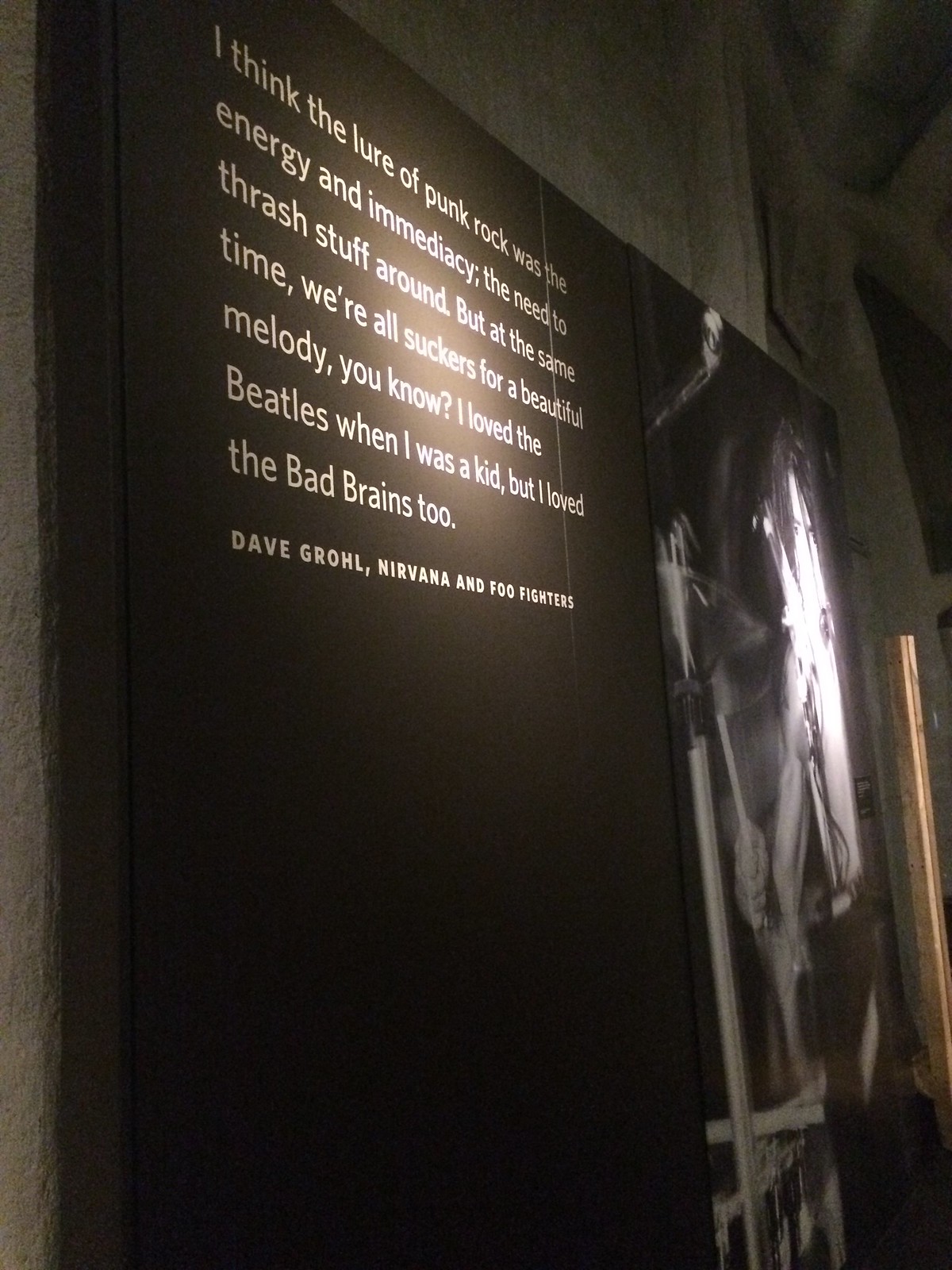The image appears to be taken at a museum, showcasing a minimalist exhibition wall. The wall has a black section with white text illuminated from above, creating a stark contrast with the surrounding white and concrete surfaces. From the vantage point, the wall's black background displays a prominent quote: "I think the lure of punk rock was the energy and immediacy, the need to thrash stuff around, but at the same time, we're all suckers for a beautiful melody, you know? I loved the Beatles when I was a kid, but I loved the Bad Brains too." This quote is attributed to Dave Grohl, known for Nirvana and Foo Fighters. 

On the right side of the wall, partially visible from the angled side view, there seems to be a black-and-white photo of a drummer, possibly Dave Grohl, striking cymbals. The lighting accentuates the photo, though the details are somewhat obscured due to the side-angle perspective of the shot. The exhibit likely celebrates elements of punk rock and may be part of a museum dedicated to music history, such as a museum of pop culture or rock music.